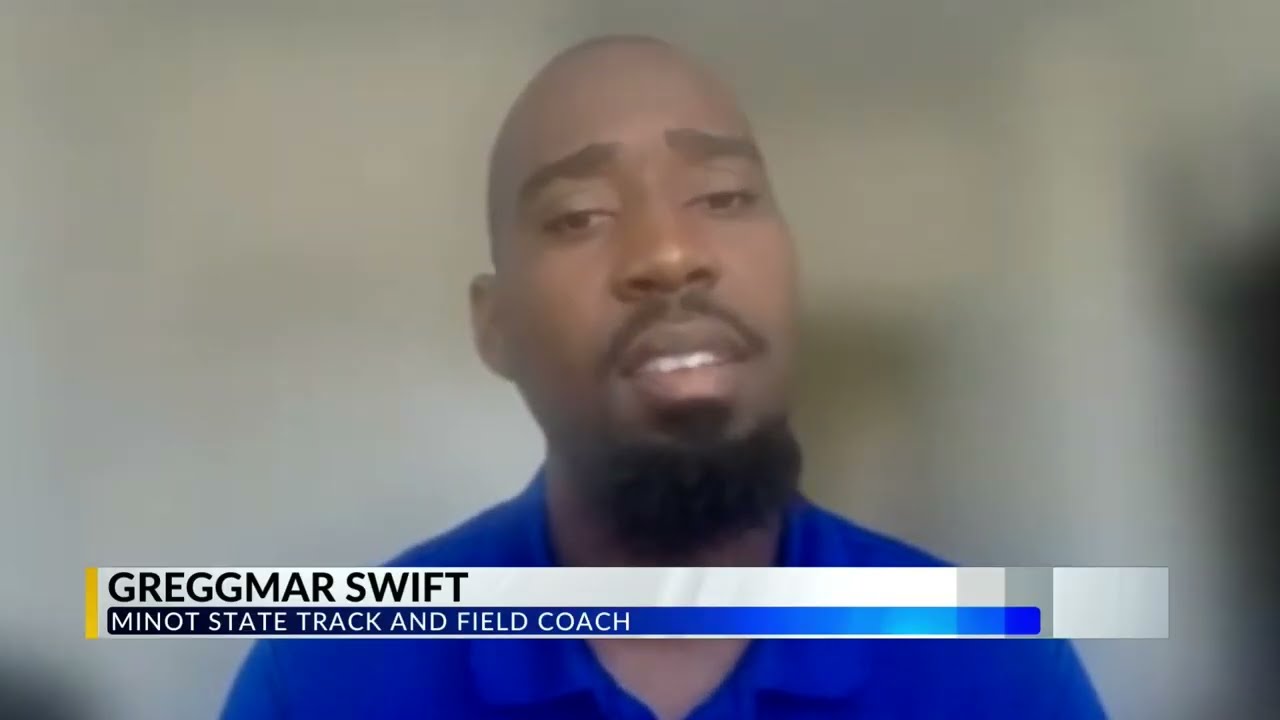The image is a color photograph of a man, evidently a still frame from a news broadcast or interview. The man, who is likely an African American named Gregmar Swift, is visually centered and occupies most of the screen from the shoulders up. He has a distinctively bald head, thick eyebrows, a mustache, and a short beard confined to his chin, giving him a bald and bearded appearance. He wears a vibrant blue collared shirt and looks directly at the camera, with a slightly open mouth suggesting he is in the midst of speaking, and his head is subtly tilted to the left, displaying a confused or concerned expression. The background of the image is entirely blurred, hinting it might be a Zoom call or some similar video setup. At the bottom of the screen, a chyron displays his name "Gregmar Swift" in black letters on a white background. Below that, in white letters on a blue bar, it says, "Minot State Track and Field Coach," and these bars extend across the lower part of the image, indicating his identity and role.